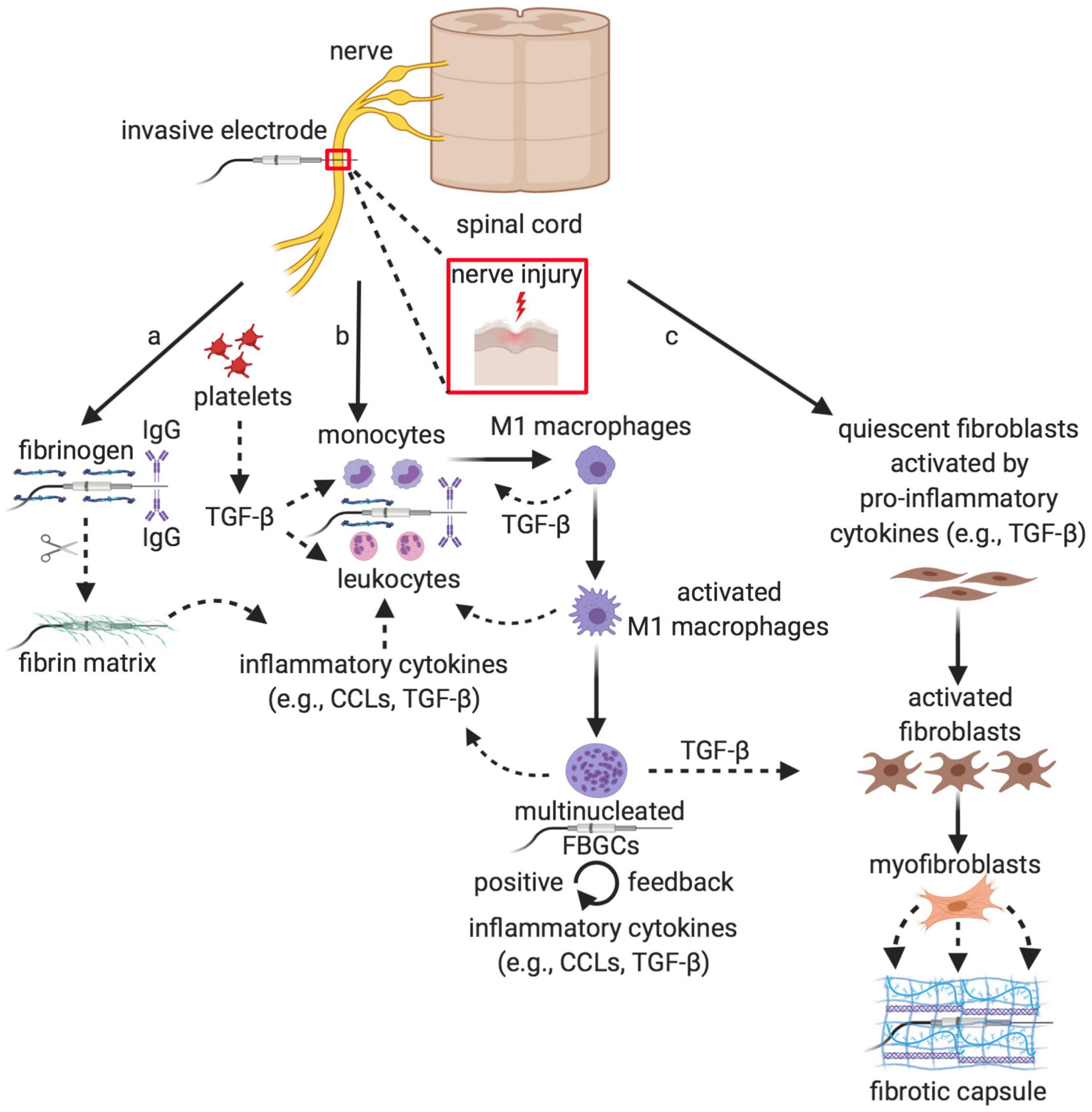This scientific diagram illustrates the effects of an invasive electrode on the nerves of the spinal cord, particularly in the context of a nerve injury. At the top, it portrays an image of the spinal cord with arrows pointing in various directions to demonstrate the process by which the invasive electrode impacts the nerves. The nerves are depicted in yellow, while the invasive electrode is marked in green, situated centrally in the image. Notable is a red box indicating areas of nerve injury. The diagram is divided into sections labeled A, B, and C, each elucidating different aspects of the impact, including the presence of platelets and the fibrin matrix, monocytes, leukocytes, inflammatory cytokines, and M1 macrophages. The actions of activated macrophages and multinucleated foreign body giant cells (FBGCs) with positive feedback mechanisms are also highlighted. The sequence progresses through fibroblasts activation leading to the formation of a fibrotic capsule, underscoring a complex cause-and-effect relationship at the site of spinal cord injury.